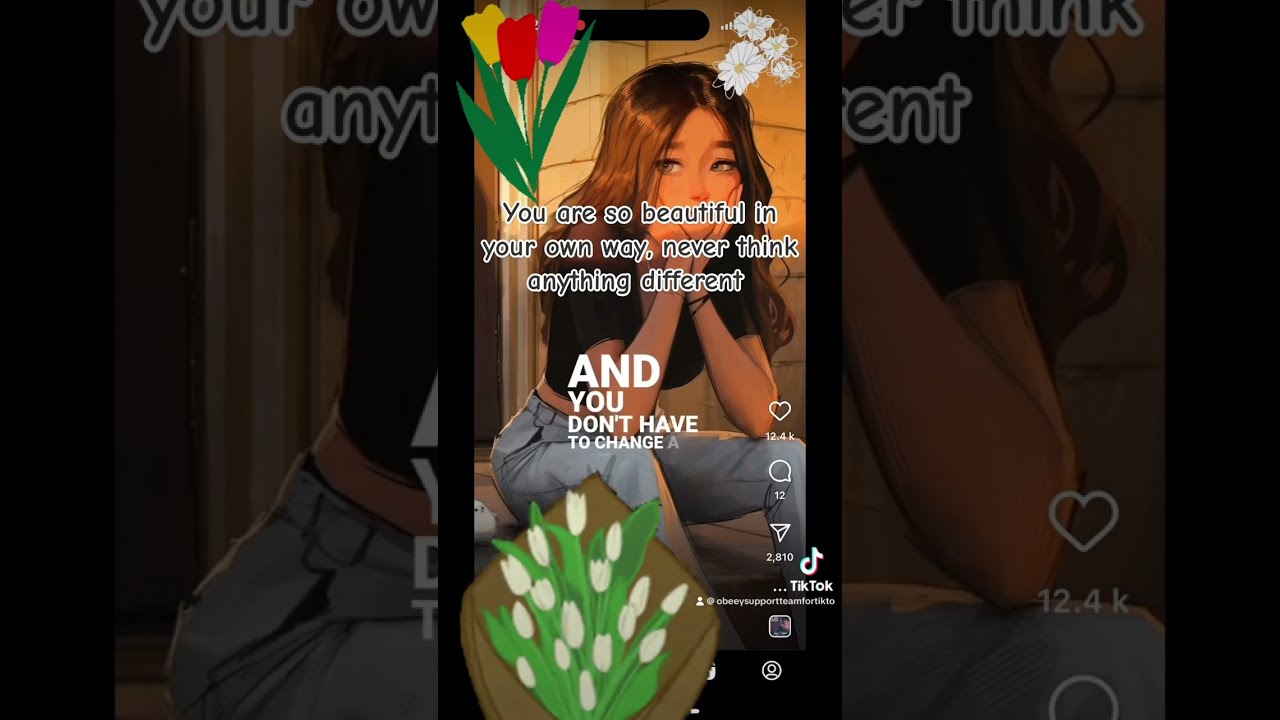The image is a screenshot of a TikTok video featuring a drawing of a young girl seated with her elbows resting on her knees and her chin nestled in her hands. She has long brown hair parted in the center and light-colored eyes gazing off to the left. She wears a black shirt and jeans. Overlaid text in a black and white bordered font reads, "You are so beautiful in your own way. Never think anything different. And you don't have to change." At the top left, there is an arrangement of red, yellow, and pink flowers with green leaves, while the top right shows only the white flower tops. In the bottom section, there's a box with white tulips and green leaves. The TikTok interface elements are also visible, including the TikTok logo, account name, and icons for liking (with 12.4K likes), commenting (with 12 comments), and sharing (with 2,810 shares). The borders of the image are heavily tinted and display enlarged, faded portions of the central image to create a background effect.